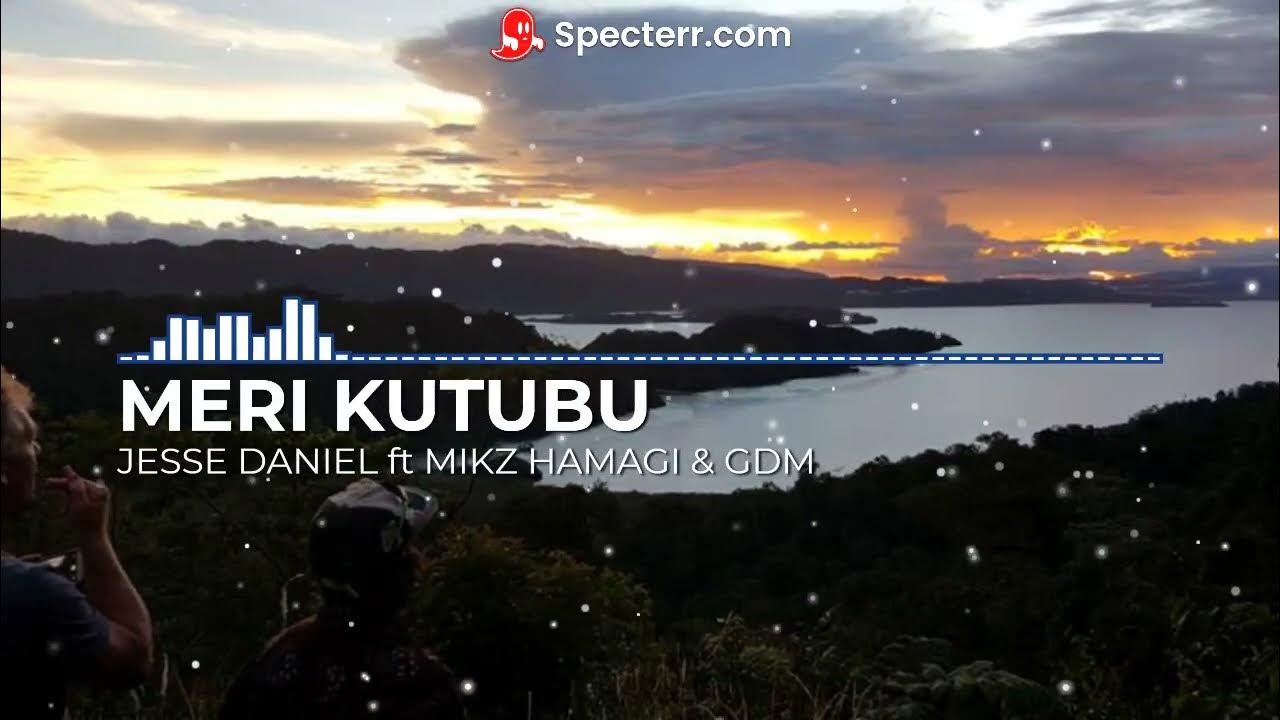The photo captures a breathtaking landscape viewed from atop a hill, bathed in the warm hues of a setting sun. In the lower left corner, a man stands, partially silhouetted against the fading light, gazing towards the tranquil lake that stretches across the middle of the image. This lake, calm and grey, is framed by darkened land and trees on the left and bottom sides, creating a striking contrast with the vibrant sky above. The sky is adorned with feathery clouds in shades of gray and white on the upper left, transitioning to orange and yellow tints as you move lower, where the sun is setting. Heavier cloud coverage is visible on the right, blending from gray to a brownish hue before becoming a brilliant orange and yellow near the horizon.

Overlaying this serene scene are digital elements. In the center, there’s a dashed line, white outlined in blue, resembling an equalizer or bar graph. Associated text below reads "Mary Kutubu" and "Jesse Daniel FT MIKZ Hamagai and GDM" in all white. At the very top center of the image, a small red Pac-Man ghost appears next to the text "Specter.com" written in white. This blend of natural beauty and digital graphics creates a unique and compelling visual narrative.